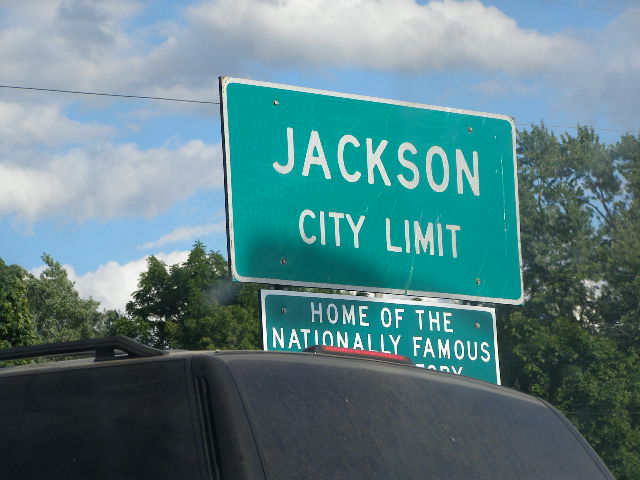The image captures a green jade rectangular highway sign that reads "JACKSON CITY LIMIT" in bold, white capital letters with a white outer lining. Below it is a partially obstructed sign that says "Home of the Nationally Famous," cut off by a black SUV with dirty, heavily tinted windows. The SUV's brake light, positioned near its roof rack, is illuminated. The scene is set against a backdrop of tall, dense green trees under a blue sky dotted with white clouds. A faint horizontal line, possibly from an electric pole, is also visible. The photo is likely taken from inside a car, adding a sense of immediate travel into Jackson, presumably Jackson, Mississippi.